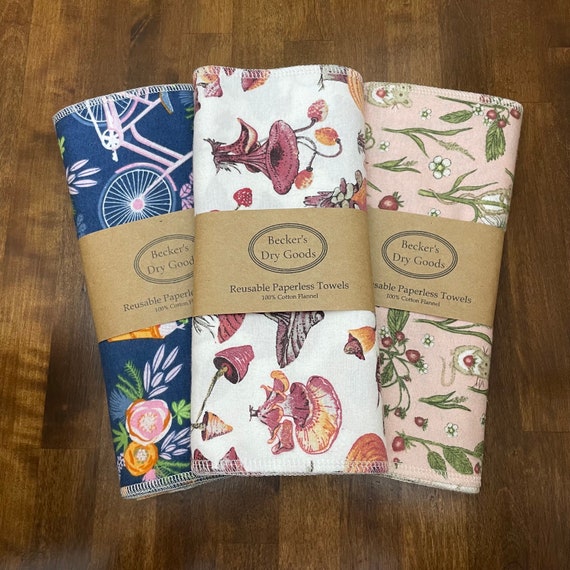The image showcases three reusable paperless towels made of 100% cotton flannel, neatly folded and rolled with a brown paper label wrapped around their center. The label reads "Becker's Dry Goods" and features three black lines, along with "Reusable Paper Towels" and "100% Cotton Flannel" written in black letters. These towels are displayed on a reddish-orange-brown stained wooden table, highlighting the wood grain and plank details. Each towel also has surged edges to prevent fraying. The first towel on the left is blue adorned with pink and yellow flowers alongside a pink bicycle. The middle towel is white with pink tulip-like flowers and pink and yellow mushrooms. The towel on the right is pink with green stems and leaves, featuring tiny strawberries.